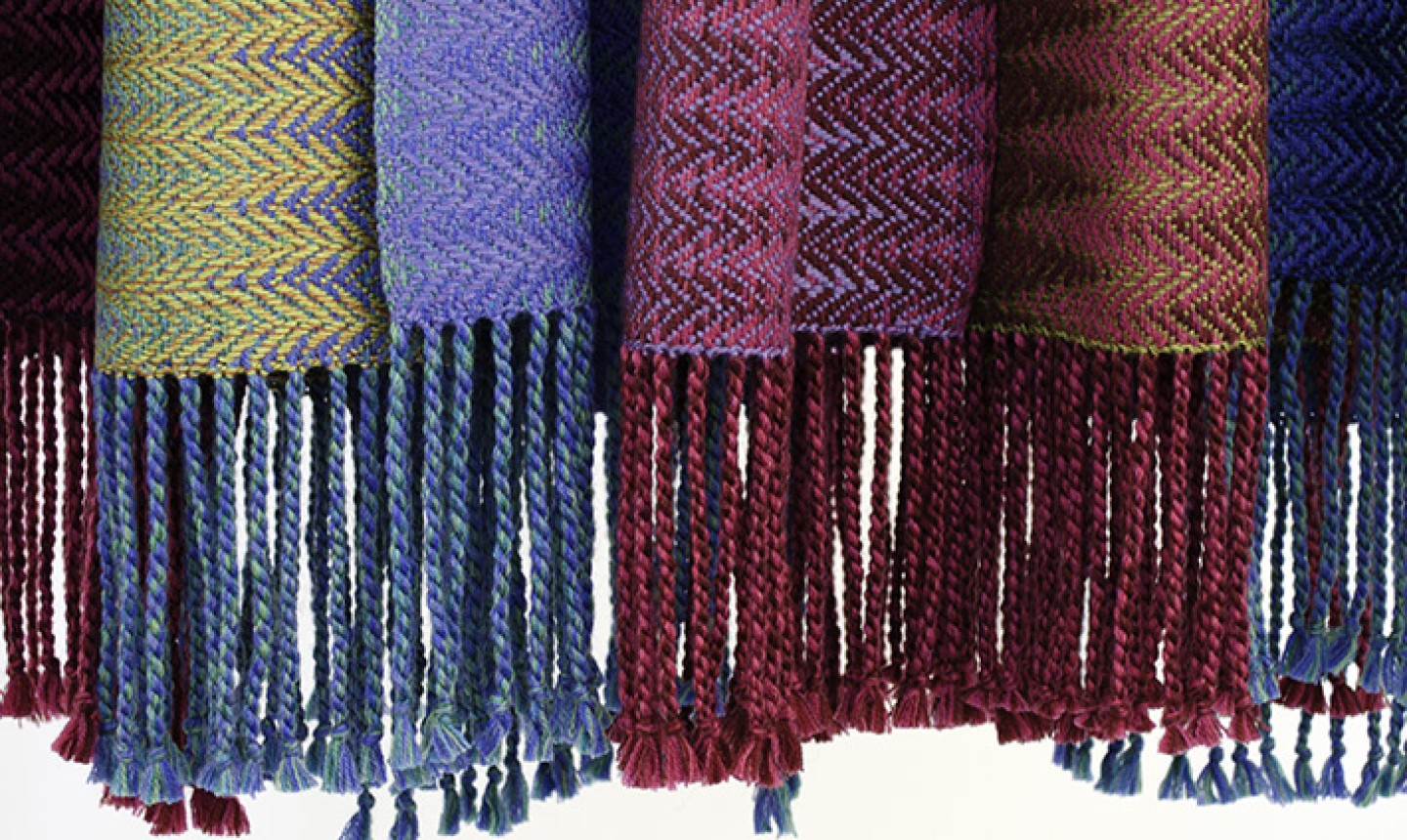This close-up photograph showcases an array of richly textured, woven fabrics, each adorned with intricate fringes dangling from the bottom. The fabrics, which could be scarves or perhaps rugs, exhibit a captivating blend of colors and patterns. Starting from the left, we see a fabric in dark purple mixed with light purple hues, followed by one with intertwined yellow and blue threads. Next comes a mix of blue and dark purple, followed by a vibrant lime green interwoven with deep dark purple. On the right end, a fabric in blue appears with hints of green and purple, suggesting a subtle, overlapping pattern. The vertical rows of woven material display a distinct V-shaped knitting pattern, blending seamlessly into each other. The fringing, made of thin yarn strips approximately 3-4 inches long, adds an elegant, flowing texture to the bottom edge of each piece. This ensemble, set against a clean white background, highlights the variety in width and length of each fabric, with certain pieces standing out more prominently than others.